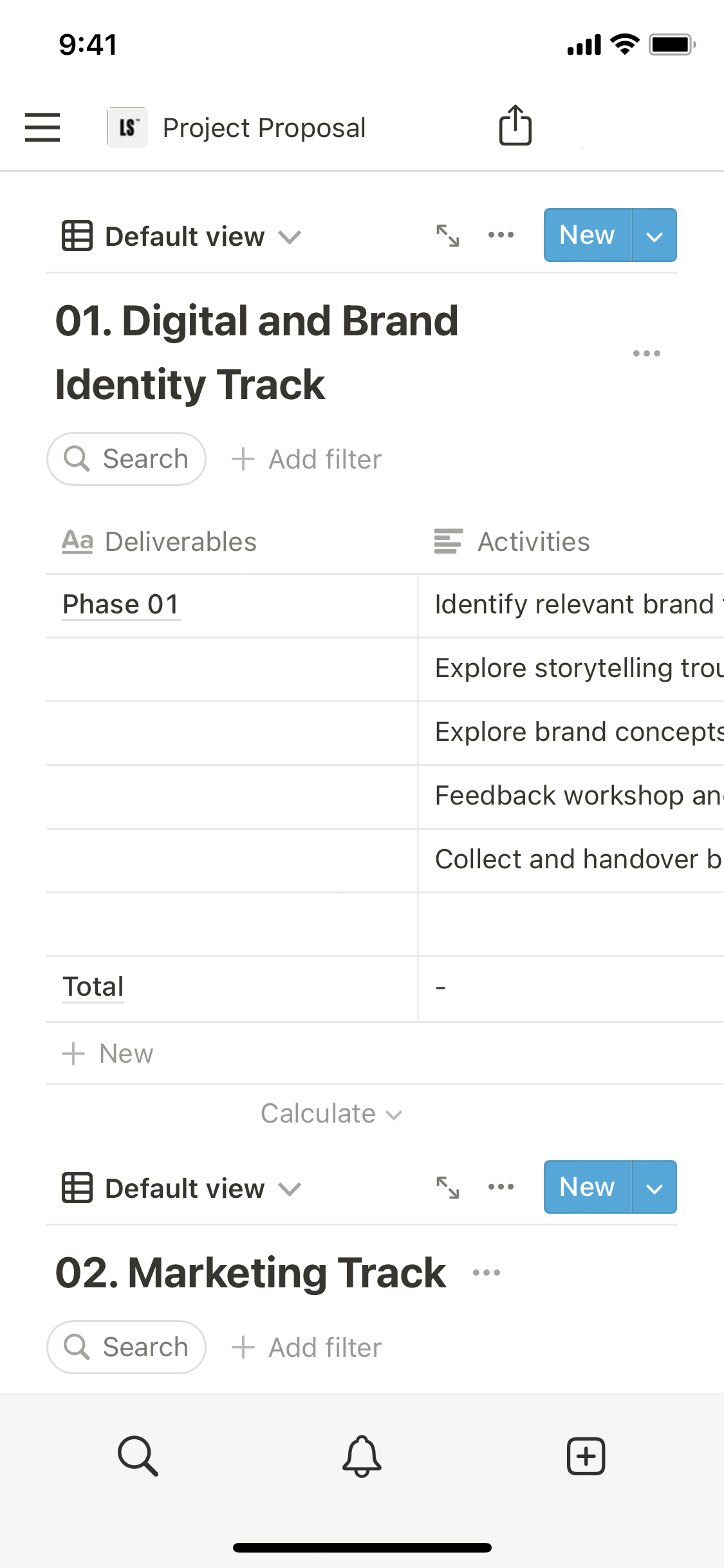In the image, the top section displays the number "941" along with four status bars. The screen also shows several labels and icons, including items like "Low Wi-Fi," "Low Boundary," "Hardware Command Units," and "Project Proposal." Various elements such as "Square," "Up-Arrow," "Default View," "New," and "C01" are scattered across the interface.

The image also showcases a section dedicated to "Digital and Brand Identity Tracking" with a search option and a "High Filter" button. Featured prominently are headings like "Deliverables," "Phase 1," "Activities," and categories such as "Identify," "Relative Brand," "Explore Storytelling," "Explore Brand Concepts," "Payback Workshop," and "Collected Handover." This area contains numerous rows, indicated collectively as "a lot of rows."

Towards the bottom, there is a detailed table or list featuring terms such as "Total," "New," "Calculate," and "Default View," accompanied by navigation arrows. Additionally, specific entries like "O2 Marketing Track," "Oval," "Search," "High Filter," "Magnifying Glass," "Bell," and "Square Plus" are mentioned. At the very bottom of the image is a grey bar, which appears slightly darker than the rest of the bottom section.